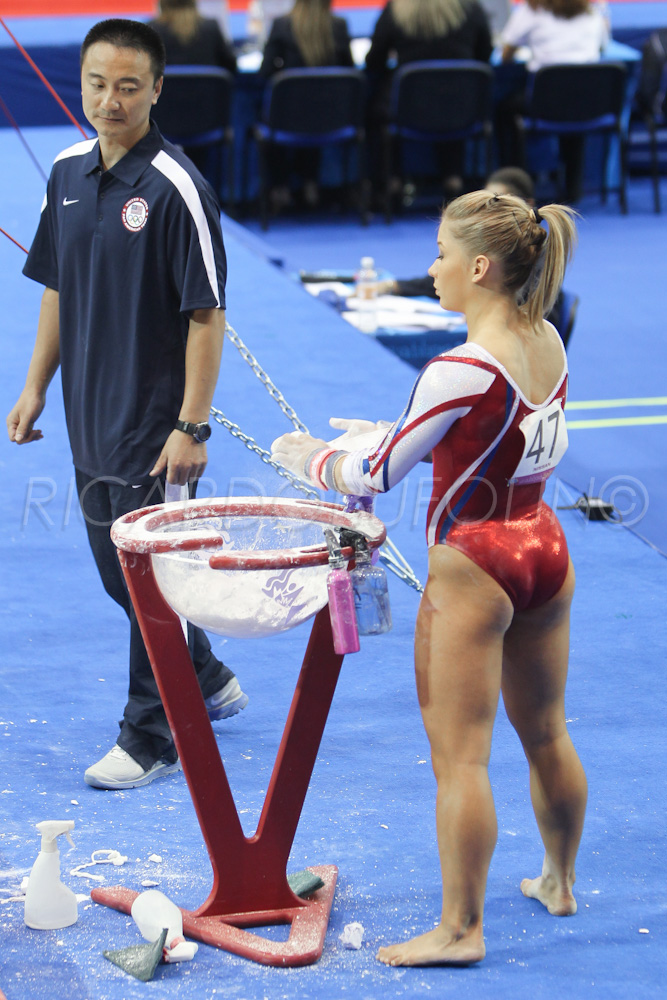In this detailed photograph, we're clearly at a gymnastics event, most likely the Olympics, given the identification on the man's shirt. The focal point is a young blonde gymnast, possibly of shorter stature, and likely Shawn Johnson, though this is uncertain. She is dressed in a striking red and white leotard with long sleeves, accented by crisscrossed red and blue stripes along the arms and sides. The gymnast bears the number 47 on her outfit and appears to be preparing for a routine, chalking up her hand guards with powder from a clear bowl on a red stand.

Accompanying her is an Asian man, perhaps her coach or a spotter, standing to her left. He is clad in dark blue pants and white shoes, with a dark blue polo shirt featuring a white stripe on the shoulder and a Nike logo on the left side. He wears a watch on his left wrist and is attentively observing the gymnast.

The gym's floor is entirely blue, and behind them is a white sign displaying black letters and the number 47. Additional details include several spray bottles scattered on the floor and hanging on the chalk stand. There are chairs in the background with people seated. The photograph is credited to photographer Ricardo Buffon, as indicated by the superimposed text on the image.